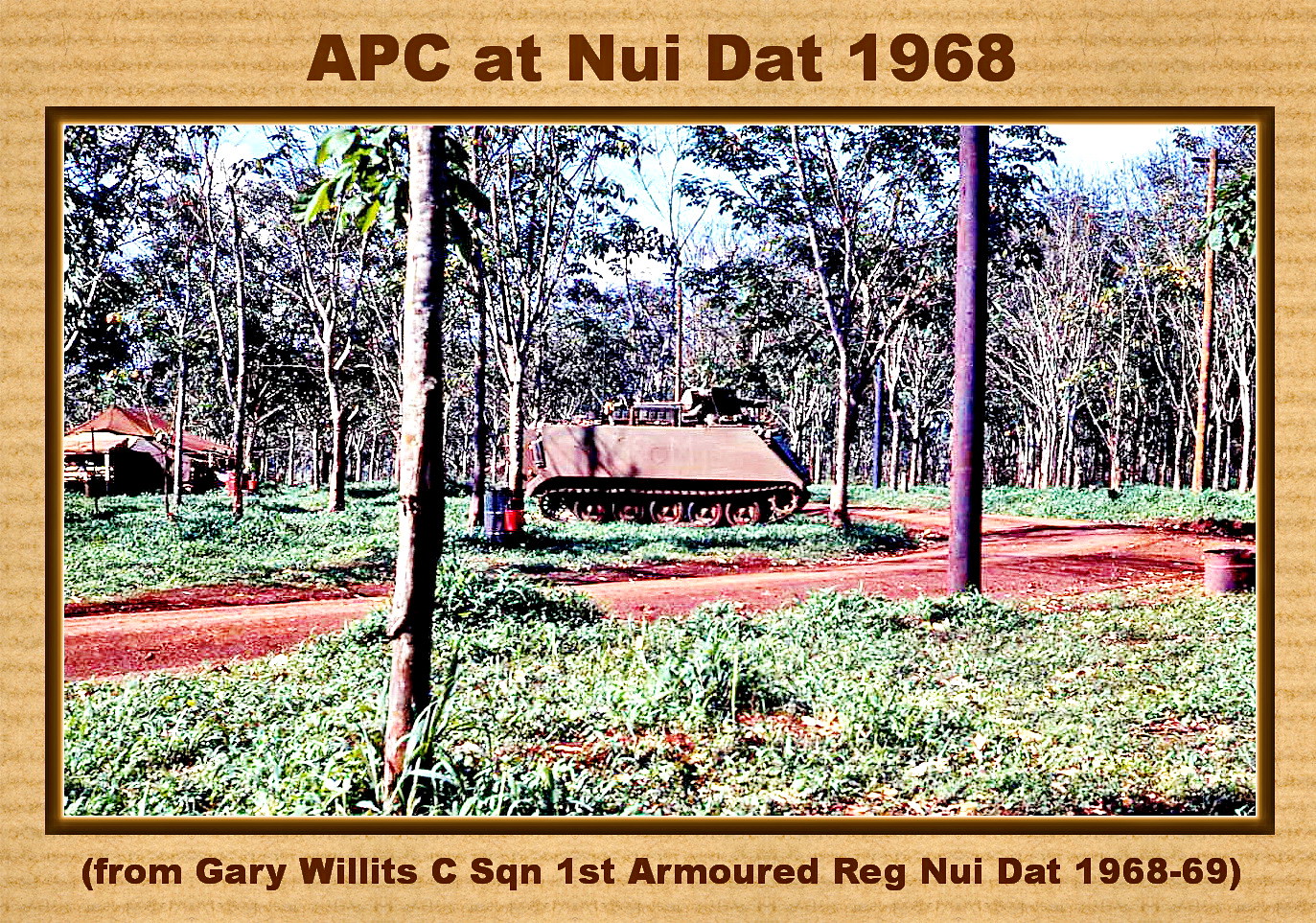The image depicts a scene from the Vietnam War, specifically from Nui Dat in 1968. The photograph features a dark brown frame with a beige matting. At the top of the image, in brown lettering, the caption reads "APC at Nui Dat, 1968," and beneath the photo, additional text in brown letters within parentheses states "From Gary Willits, C-Squad, 1st Armored Regiment, Nui Dat, 1968-69."

In the center of the scene, an armored personnel carrier (APC) is prominently displayed, equipped with a mounted machine gun. The APC is positioned on the side of a red dirt road that curves to the left. The foreground shows sparse, scrubby grass while in the background, a dense jungle is visible, although the immediate area around the APC and road has fewer trees. Off to the left side of the image, slightly behind the APC, there is an old, rundown Japanese shack partially hidden by the foliage. The entire scene is devoid of human presence, creating a stark, empty atmosphere in the midst of the jungle setting.